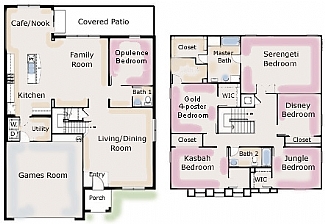This two-story house blueprint features an array of thoughtfully designed spaces. The main level includes a cozy café nook, a covered patio for outdoor relaxation, and a spacious family room. Adjacent to the family room is an opulent bedroom complete with an en-suite bathroom. On the opposite side, you'll find the kitchen and a utility room. Beyond the kitchen lies a game room, which boasts an attached porch - doubling as the primary entrance to the home - leading directly into the living room.

The second floor hosts several uniquely themed bedrooms. There is a Disney bedroom with just a closet, a jungle-themed bedroom inclusive of its own bathroom, and a Cosby bedroom adjacent to a bathroom with its own closet. Additionally, there is a luxurious gold four-poster bedroom, also featuring a private bathroom. The highlight is the master bedroom, known as the Cerganti bedroom, which comes with an en-suite master bathroom. Centrally located among these rooms are stairs that lead up from the main level. For convenience, there is also a shared bathroom accessible to the bedrooms that do not have private facilities.